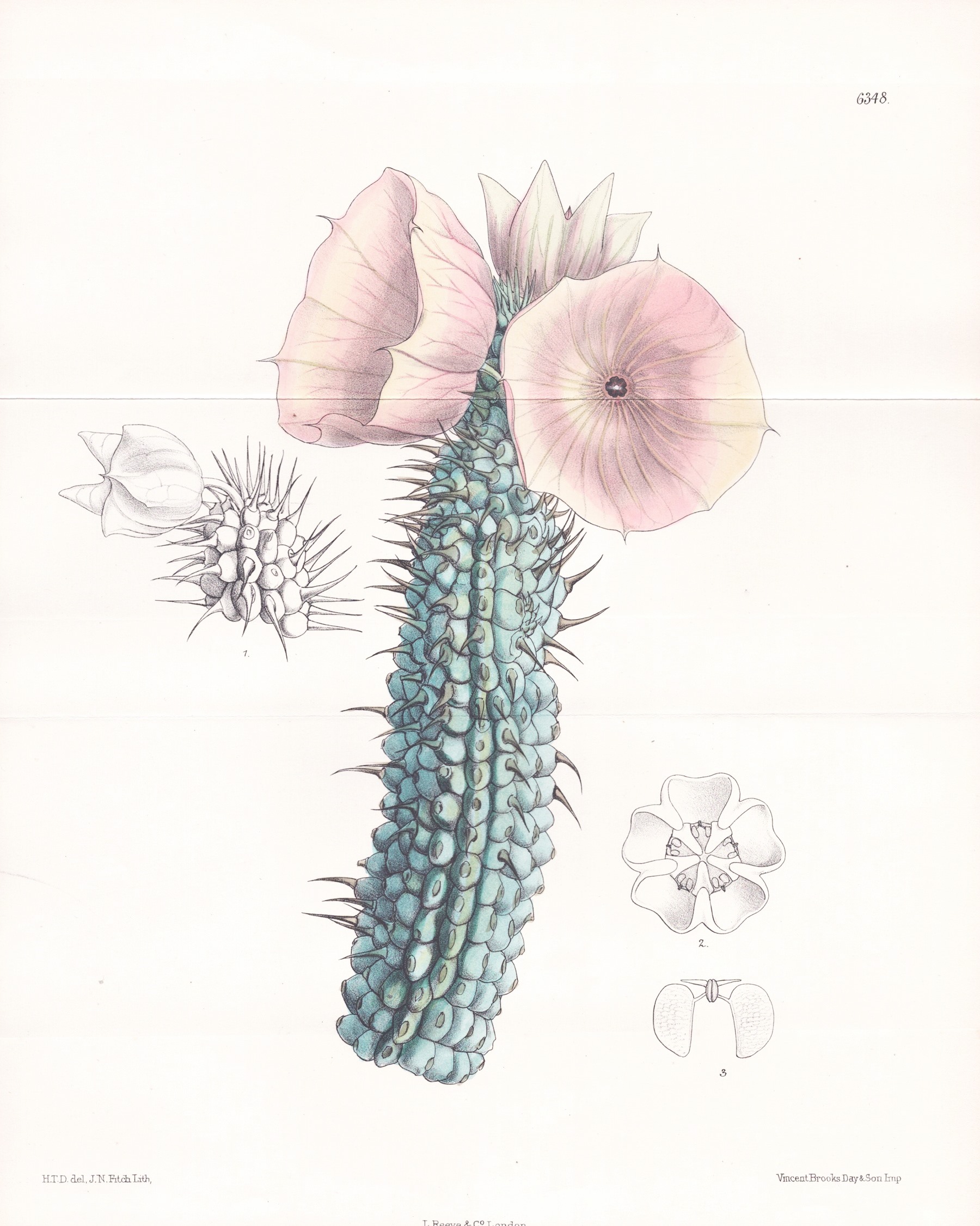This image, which resembles an illustration from a textbook, features a detailed depiction of a unique plant that extends vertically from bottom to top, centered within the frame. The plant's stem is distinctively blue and adorned with blackish spikes. As the stem ascends, three flowering blooms emerge at the top. These flowers have delicate pink and white petals with pointed tips forming a circular pattern, reminiscent of moon flowers.

The image rests on a piece of paper with a light pinkish background, measuring approximately 6 inches in height and 4 to 5 inches in width. A horizontal fold is present about an inch and a half from the top. Noteworthy details include a small black print reading '6348' in the upper right corner and additional printed text in the lower left and right corners, along with a third piece of text cut off at the bottom. This text includes watermarks such as ‘HTD Del’ and ‘Vincent Brooks Day and Son Imp.’

Adjacent to the central plant, the illustration features black and white drawings on either side. On the left is an enlarged detailed sketch of a flower, while on the right bottom corner, there is an illustration showing the petals in black and white, alongside a quick internal sketch of the floral structure. The combination of colored and monochrome elements provides an in-depth botanical study, enhanced by the meticulous details of both the main plant and its components.